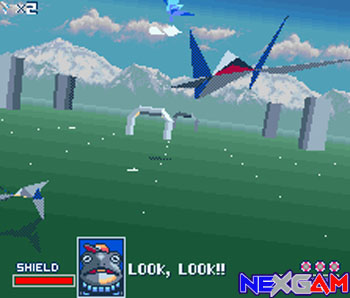This image is a slightly pixelated screenshot from the video game Star Fox, specifically resembling the first level of Star Fox 2 on the Super Nintendo. The scene is set with a blue sky dotted with clouds and a mountainous horizon in the background. The central portion of the image features two prominent arches, with the closer one being white and the further one gray. Flanking these arches are four gray columns on either side of the image.

In the upper left-hand corner, there is a symbol followed by "x2." The upper right corner showcases a spaceship with blue triangular wings and a body constructed of multiple silver triangles; another smaller gray ship is visible in the bottom left-hand corner. Additionally, a geometric plane-like object colored red, white, and blue can be seen at the top of the image.

Prominent text elements include a red bar labeled "SHIELD" and a frog cartoon character wearing a gray hat with dialogue next to it saying, "LOOK, LOOK." Finally, in the bottom right corner, there is text that spells out "NEXT GAM" in a decorative font with "N-E" in blue, "X-G" in gray, and "A-M" in red, along with three circles above the text. The overall image is slightly askew, adding to its dynamic appearance.